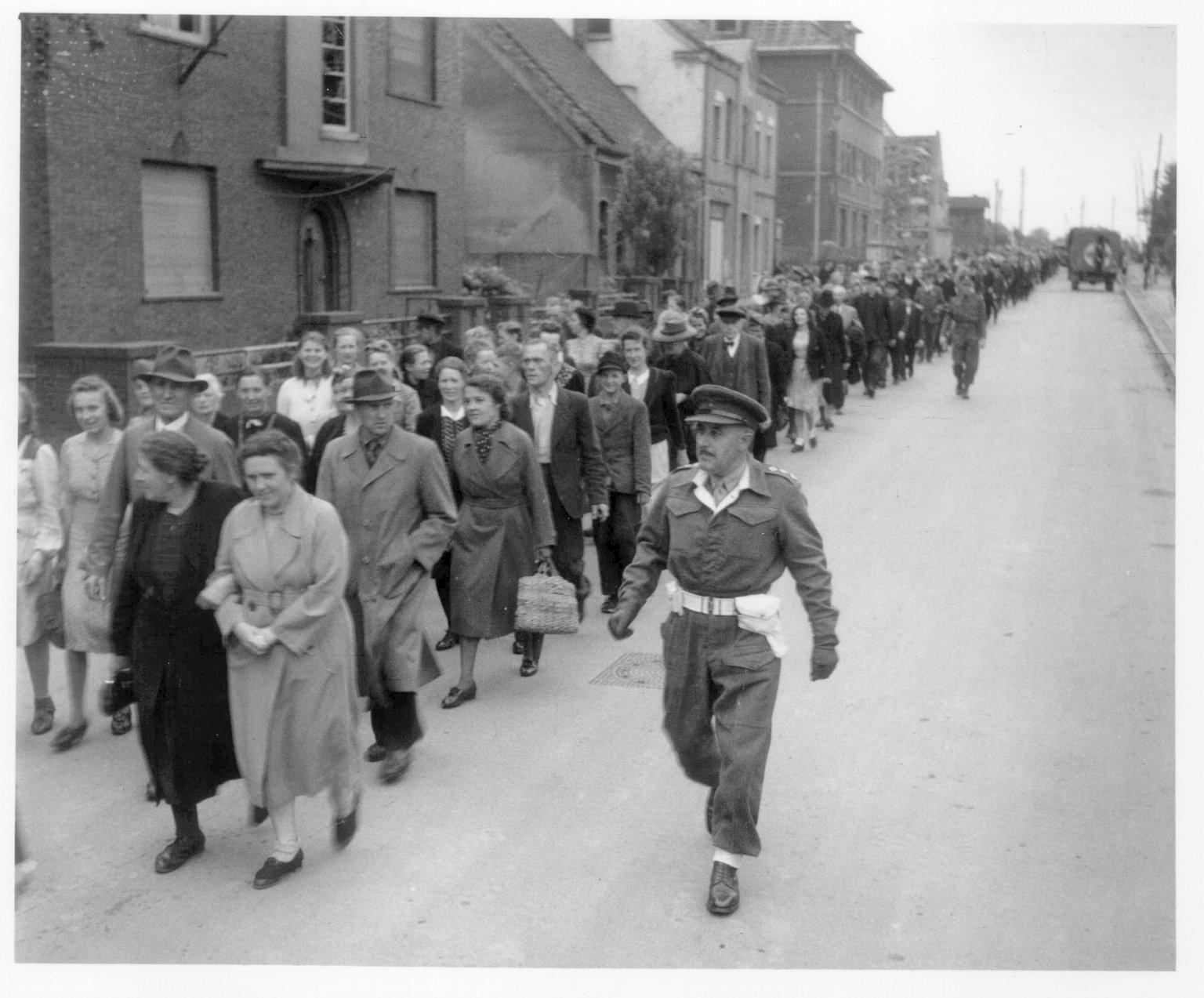In this evocative black and white photograph, a massive line of people extends from the bottom left corner of the image and stretches diagonally across the road, almost reaching the top right corner. These individuals, both men and women, predominantly dressed in jackets and trench coats, appear to be walking in unison towards a distant destination. Among them are soldiers, identifiable by their uniforms and flat caps with brims, who flank the procession, seemingly guiding or overseeing the march. The left side of the road is lined with grey-toned buildings and houses, while an army vehicle is visible on the right, further along the street. The photograph exudes a historical atmosphere, potentially from the 1930s or 1940s, and captures a moment filled with a mixture of solemnity and resilience as the crowd progresses forward.